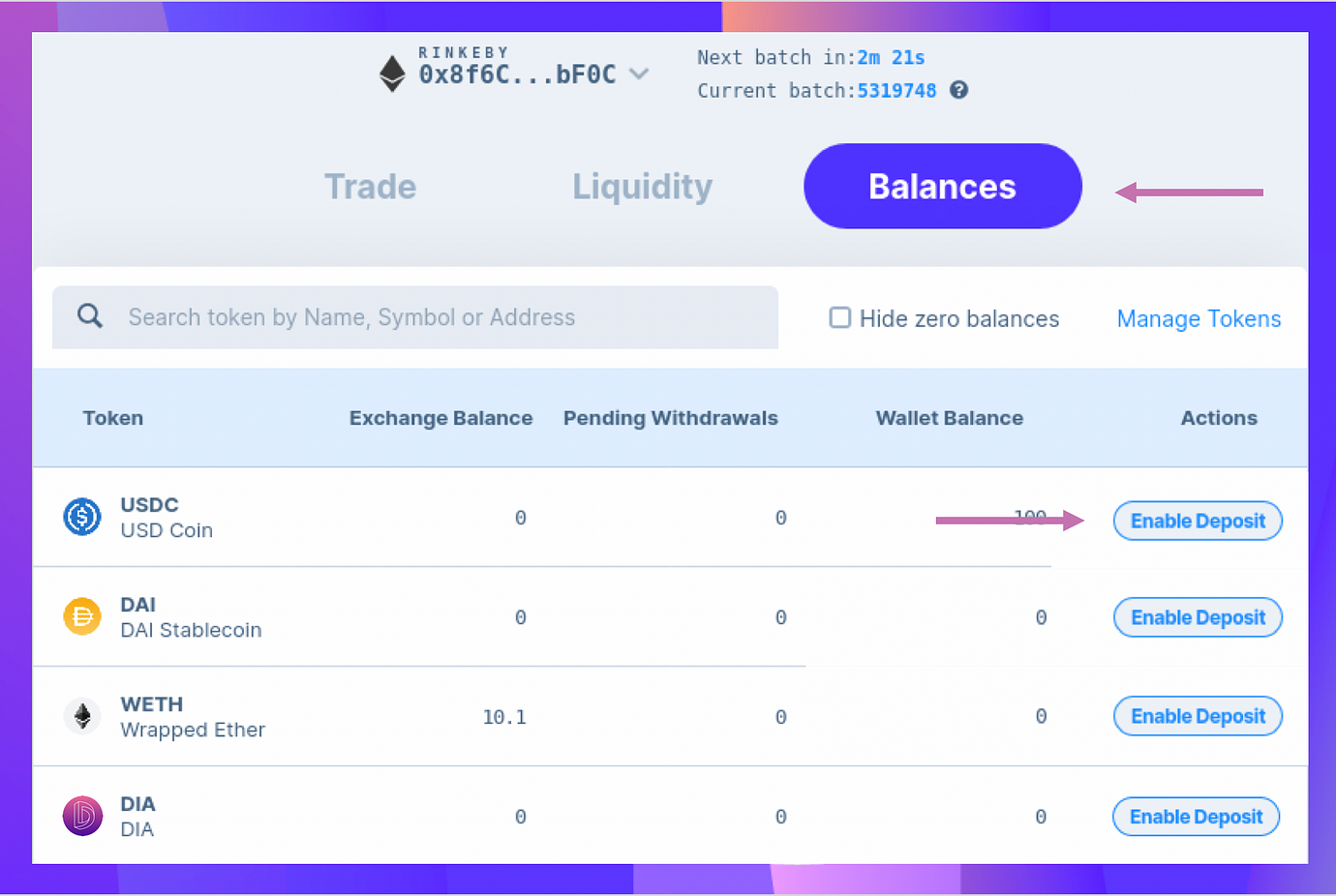This screenshot image, captured in landscape mode, showcases a digital interface with an abstract background that transitions from pink to blue, purple, and a hint of yellow. The interface content is primarily gray and white, outlined and accentuated by various highlights and pointers.

At the top center of the image, a notification displays: "RINKEBY, Next batch in 2 minutes, 21 seconds, current batch 5319748." Below this, the interface indicates a row titled "Trade Liquidity," with a blue button labeled "Balances" that is marked by a violet arrow, directing the viewer's attention to this button.

The next section features a white background with a gray search bar containing the placeholder text: "Search token by name, symbol, or address." Adjacent to this search bar, on the right side, there is a checkbox labeled "Hide zero balances." Further to the right, another blue button reads "Manage Tokens."

Directly underneath, a blue banner provides the following headings: "Token Exchange Balance, Pending Withdrawals, Wallet Balance Actions." To the left, a list of different tokens is displayed, including USDC (USD Coin), DAI (Dai Stablecoin), WETH (Wrapped Ether), and DIA (DIA).

The "Exchange Balance" column indicates zero for each token. Highlighted by a prominent pink arrow, the primary action on the first token row, labeled "USDC," involves the "Enable Deposit" option, suggesting the intended interaction.

Overall, the individual has thoughtfully marked specific elements, guiding users to interact with particular functions of this digital trading or wallet interface.